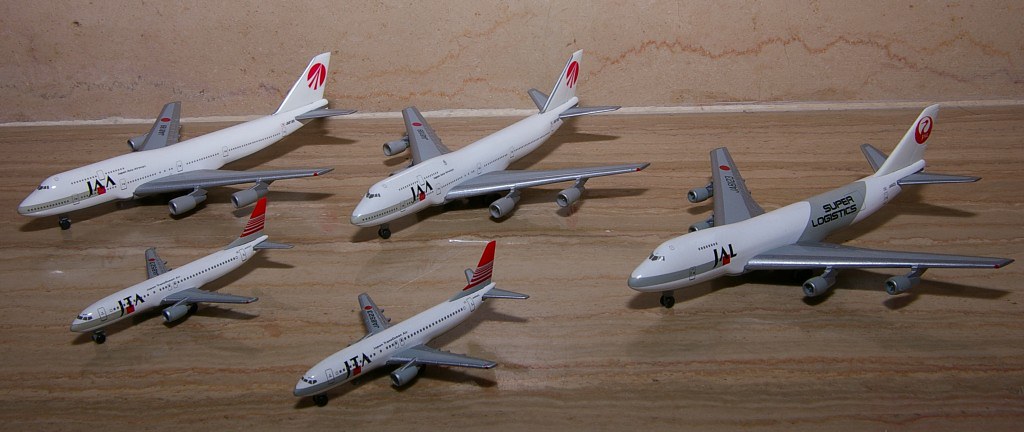This photograph showcases five model airplanes, each meticulously detailed with the same color scheme and logos, specifically JAA, JTA, and JAL. Arranged on a wooden counter with a distinct, marbled tile background in shades of brown and pink-orange, these model airplanes vary in size and design. The larger models, positioned at the top, exhibit intricate features including four jet engines, while the smaller ones at the bottom display fewer engines—primarily two—and visible passenger windows. Notably, one of the larger models bears the label "Super Logistics," distinct for its lack of windows, indicating it's not a passenger plane. All models feature a predominantly white body with red tails and silver wings, capturing the essence of a cohesive fleet despite their varying designs and purposes.